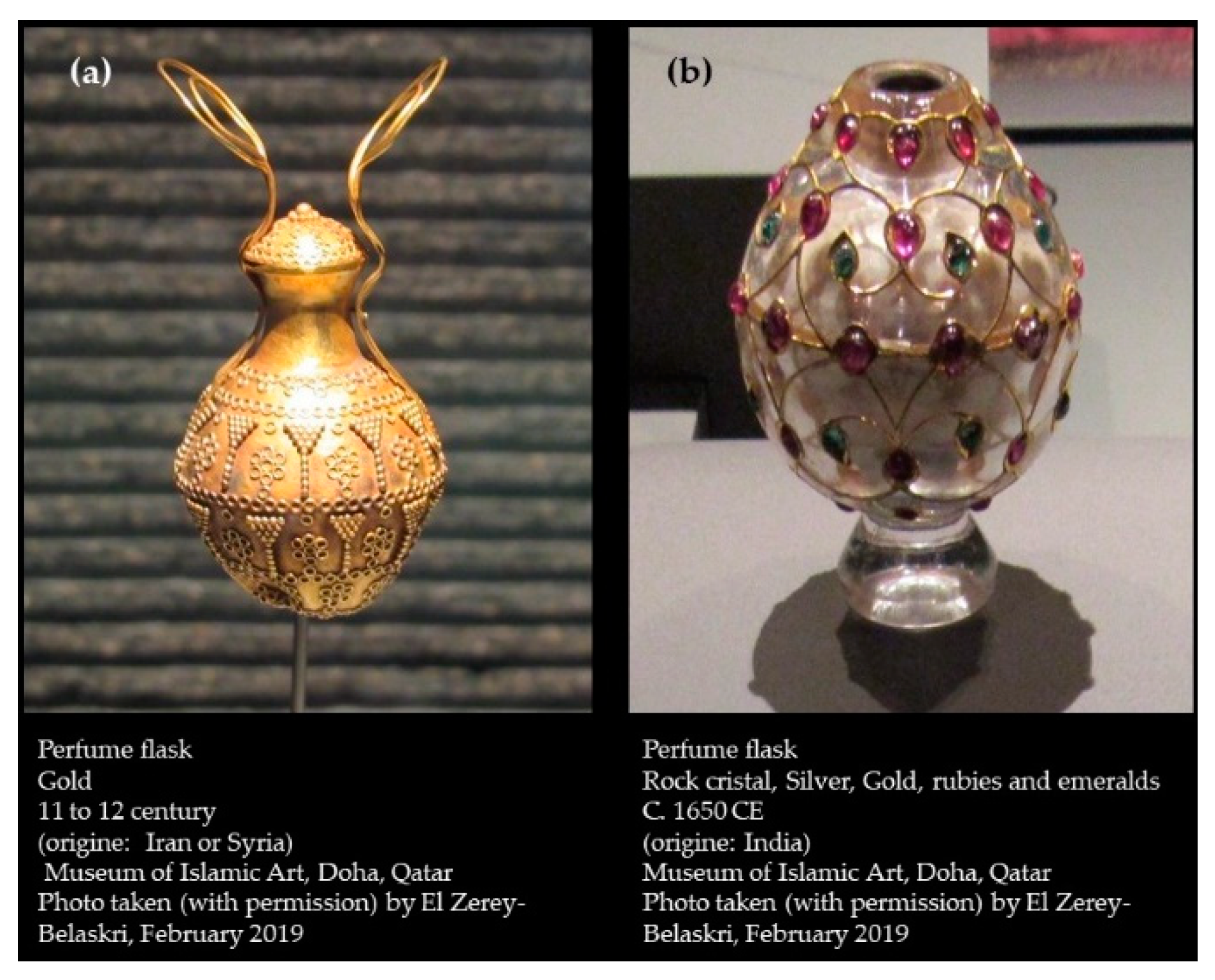The image displays two side-by-side photographs of ornate perfume flasks, each accompanied by detailed descriptions. On the left, labeled as 'A', is a gold perfume flask from the 11th to 12th century, originating from Iran or Syria. This intricately designed flask features a large base and a closing mechanism at the top. The text beneath this image reads, "perfume flask, gold, 11th to 12th century, origin Iran or Syria, Museum of Islamic Art, Doha, Qatar," with the photo taken by El-Zeray Belaskri in February 2019. On the right, labeled as 'B', is a luxurious perfume flask composed of rock crystal, silver, gold, rubies, and emeralds, dating back to circa 1650 CE from India. This flask, with its pearl and glass-like texture and ornate gold designs adorned with various gemstones, appears to rest on a table. The accompanying text states, "perfume flask, rock crystal, silver, gold, rubies, and emeralds, circa 1650 CE, origin India, Museum of Islamic Art, Doha, Qatar," also photographed by El-Zeray Belaskri in February 2019. Both photographs, capturing these historical and lavish artifacts, are exhibited in the Museum of Islamic Art in Doha, Qatar.